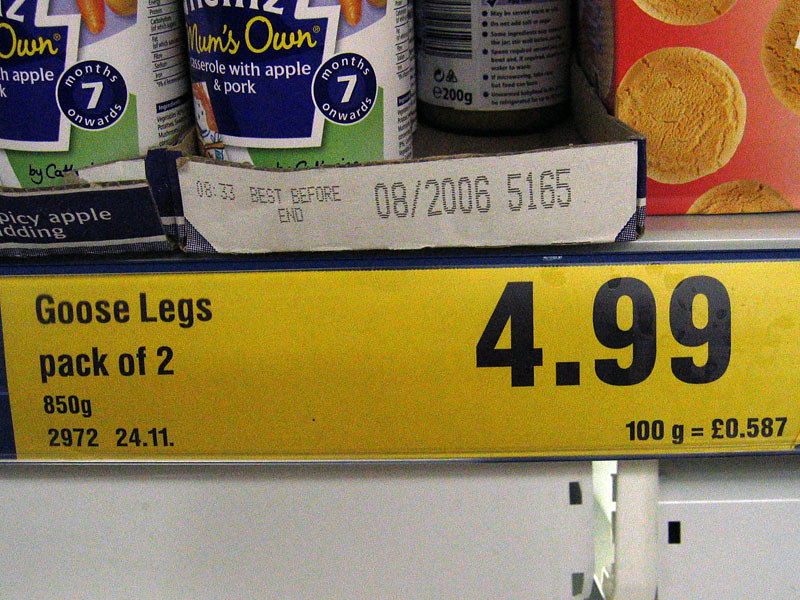The image captures a grocery store shelf packed with various food items. Prominently featured is a large, bright yellow sales label with black text that reads "Goose Legs, pack of two, 850 grams," priced at $4.99. Below the price, there is detailed information including "2972, 24.11", and "100 grams equals 0.587 pounds." In front of this label, there are containers of food, with one labeled "Spicy Apple Pudding" and another "Mum's Own Casserole with Apple and Pork." The casserole containers have an expiration date stating "best before end 08-2006-5165." To the right, a packet of biscuits, likely gingersnaps, is visible against a red and white background. Above these items, there are shelves holding canned goods including more "Mum's Own Casserole with Apple and Pork" tins. The shelf itself is metallic with holes cut into the racking, suggesting sturdy, industrial design. In the background, more store shelves and price tags can be seen, situating the scene firmly within a grocery store setting.